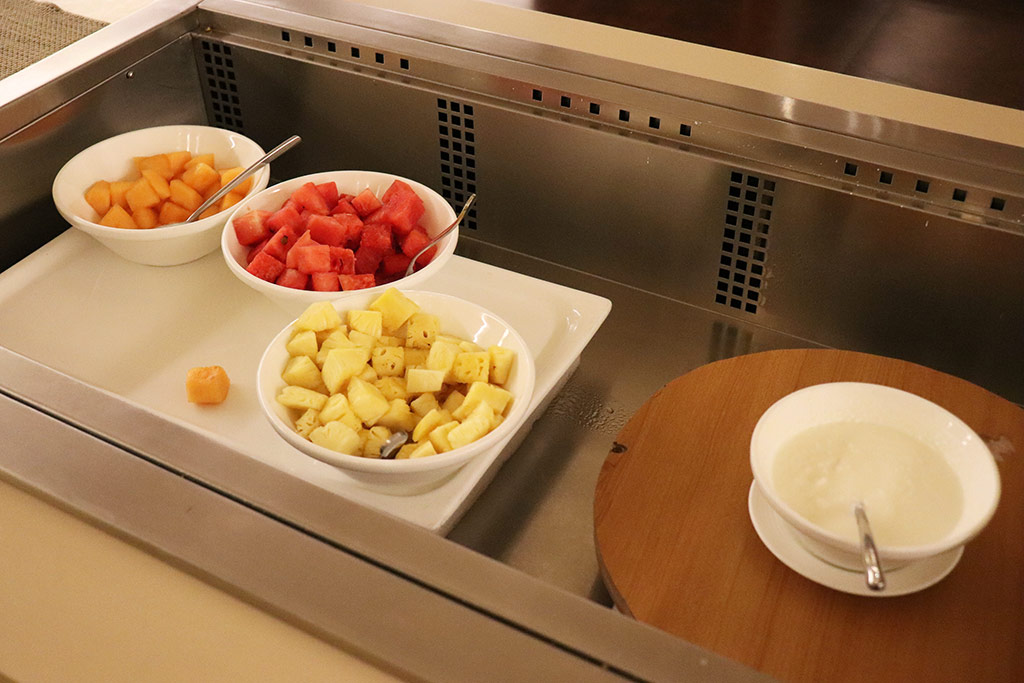In a pristinely clean kitchen preparation area, a sleek stainless steel countertop features an organized setup. At the center lies a large, white porcelain serving tray holding three distinct bowls filled with cubed fruits—vibrant orange cantaloupe, juicy red watermelon, and succulent yellow pineapple. A piece of cantaloupe has tumbled out of its bowl, adding a touch of casual imperfection to the otherwise orderly setting. Each bowl is accompanied by a unique serving spoon, hinting at the care and attention given to even the smallest details.

To the right side of this setup, a wooden circular board showcases a smaller porcelain bowl perched on a matching saucer. This bowl contains a thick, white porridge, with a spoon that appears ready for serving. The entire arrangement suggests a well-organized, professional food preparation area, possibly in a communal or commercial kitchen.